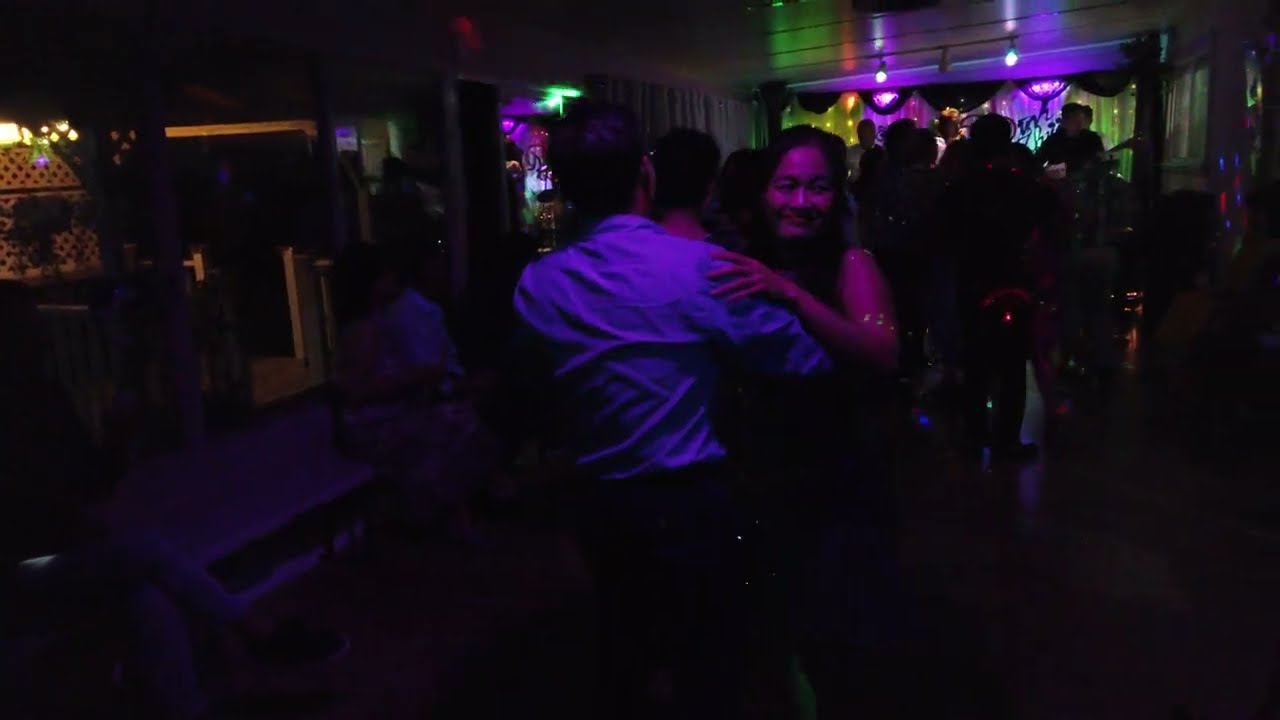In this horizontally aligned rectangular image, a dark and somewhat blurry setting suggests a club or a party atmosphere. Dominating the center frame is a dancing couple. The woman, an Asian with at least shoulder-length black hair, smiles towards the right while resting her left hand on the man's shoulder. She is dressed in a sleeveless outfit, though other details are obscured by the dim lighting. The man, seen from the back, sports short black hair, glasses, a long-sleeved blue shirt, and dark slacks. Around them, shadowy figures of people fill the background, their details blurred by the low light. Sparse illumination comes from a few ceiling spotlights in the upper part, casting purple hues, and some distant, faint white lights. The left side reveals a partially visible walkway leading to another section, while the upper left corner remains completely dark. The bottom part of the image is mostly black, hiding any details of the flooring. There are no text elements within the picture, which overall captures a faint, vibrant nightlife ambiance.